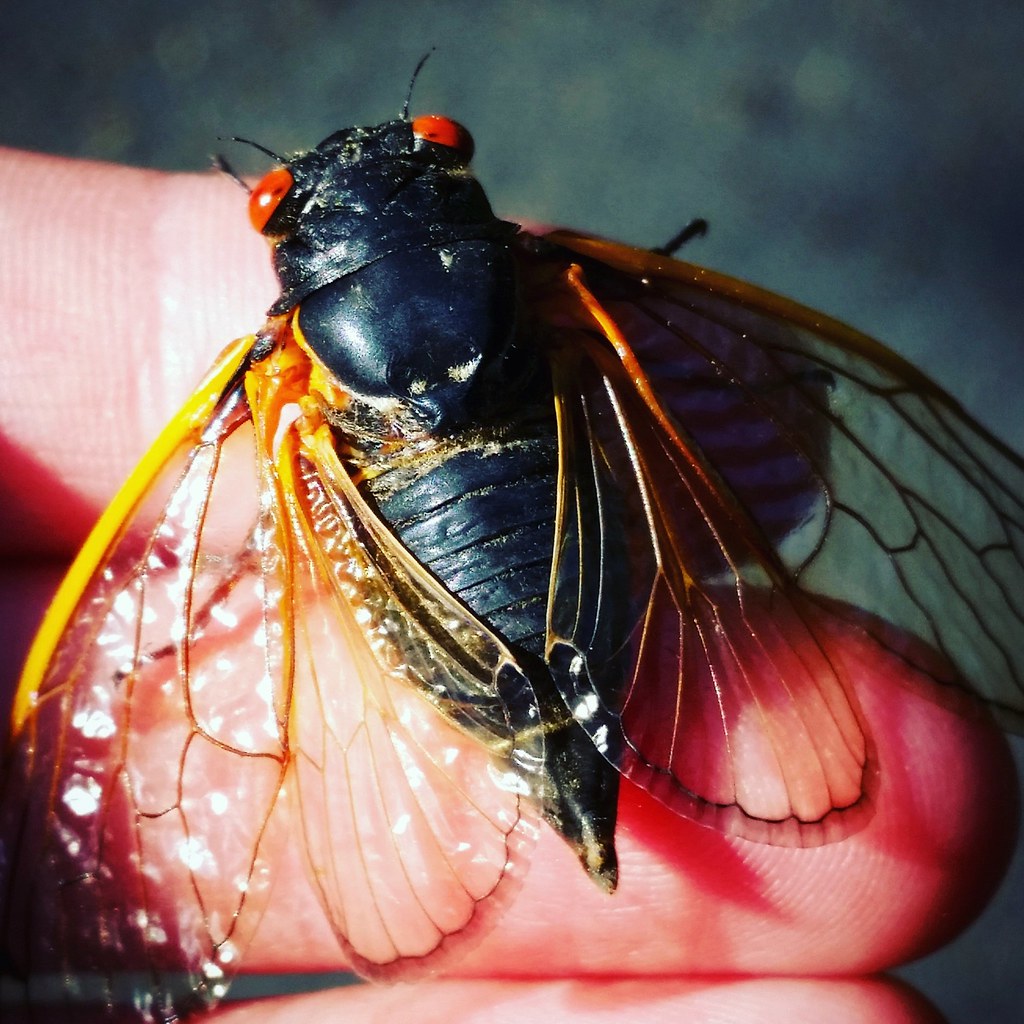This close-up, square photograph captures an intricately detailed, large black insect perched on the tips of three fingers emerging from the left side of the frame. The insect's translucent wings, which are spread out, feature distinctive yellow borders and lines. Its eyes are a notable orange-red color, contrasting sharply with its black body. The body tapers down to a very sharp point, and there's a greenish-hued background that complements the scene. The insect is about the length of two fingers, with its wings resembling delicate, almost glass-like structures. The detailed view highlights the insect's unique and fascinating physical features.